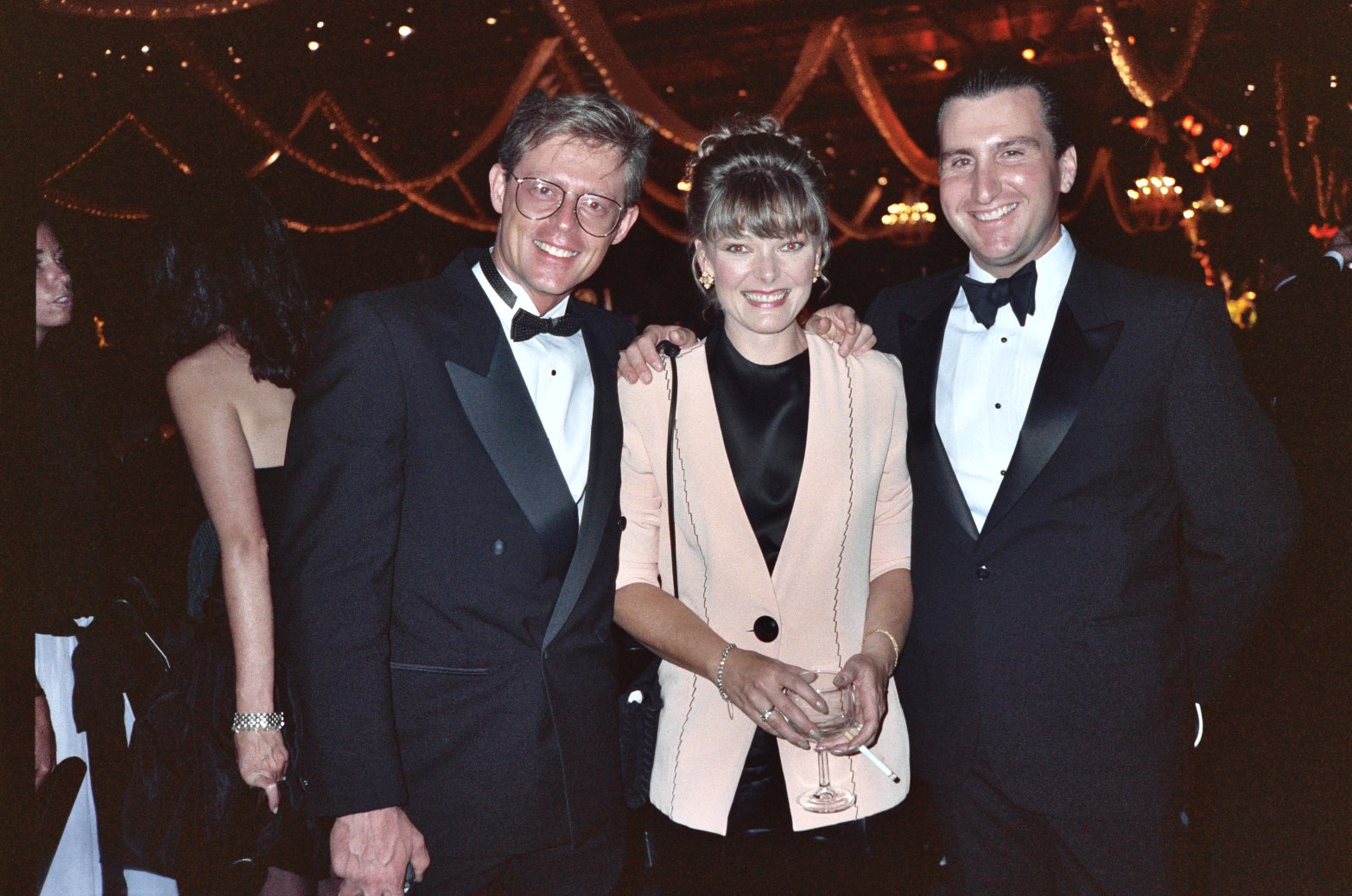The image captures a lively gathering of celebrities, likely including well-known actors and actresses. On the far right is a smiling man dressed in a classic black tuxedo with a white dress shirt and a black bow tie. He has short brown hair and an approachable demeanor. Centered in the image is a woman wearing a stylish black top with a small, fashionable jacket draped over it. She holds a glass of what appears to be an alcoholic beverage, possibly wine, while she casually smokes a cigarette. Her short brown hair is styled with bangs, and she accessorizes with elegant earrings. Adjacent to her is another man, distinguished by his glasses and similarly clad in a black tuxedo. Their backdrop features flowing red curtains, adding a touch of sophistication and warmth to the scene. In the background, more individuals contribute to the atmosphere of the event, enhancing the sense of a bustling, glamorous social gathering.